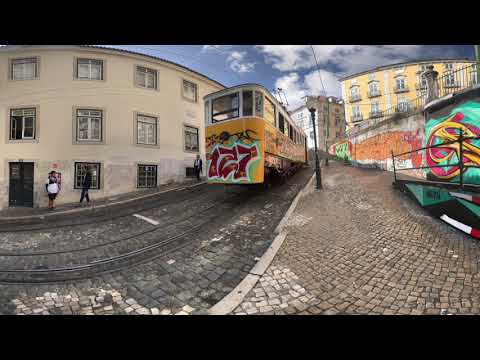The image is a detailed color photograph showing a residential area in a city, presented in a panoramic format with a black horizontal stripe across the top and bottom. The scene captures a cobblestone street with a dual rail track for a trolley train running down the middle, heading downhill towards the viewer. The trolley train, the focal point of the image, features windows at the top and is distinctly adorned with colorful graffiti art in black and red, with the number "727" prominently displayed on its yellow front. Contrasting graffiti, including hues of green and orange, is noted in the descriptions but could be a result of different perspectives in the panorama. 

On the left side of the image stands a three-story beige stucco building with rectangular windows on every floor. Near the entrance, a couple of people are seen standing around. To the right, the street is framed by a brick wall covered in vibrant graffiti. This side of the street also features a black iron handrail and black lamp posts with white lights at the top. In the background, a tall, somewhat decrepit yellow building with numerous windows is visible, lending a historical feel to the urban landscape. The sky is a clear blue with a few wispy clouds, indicating a pleasant daytime setting. The overall composition blends elements of realism and photographic representationalism, capturing the dynamic and slightly eclectic essence of the cityscape.